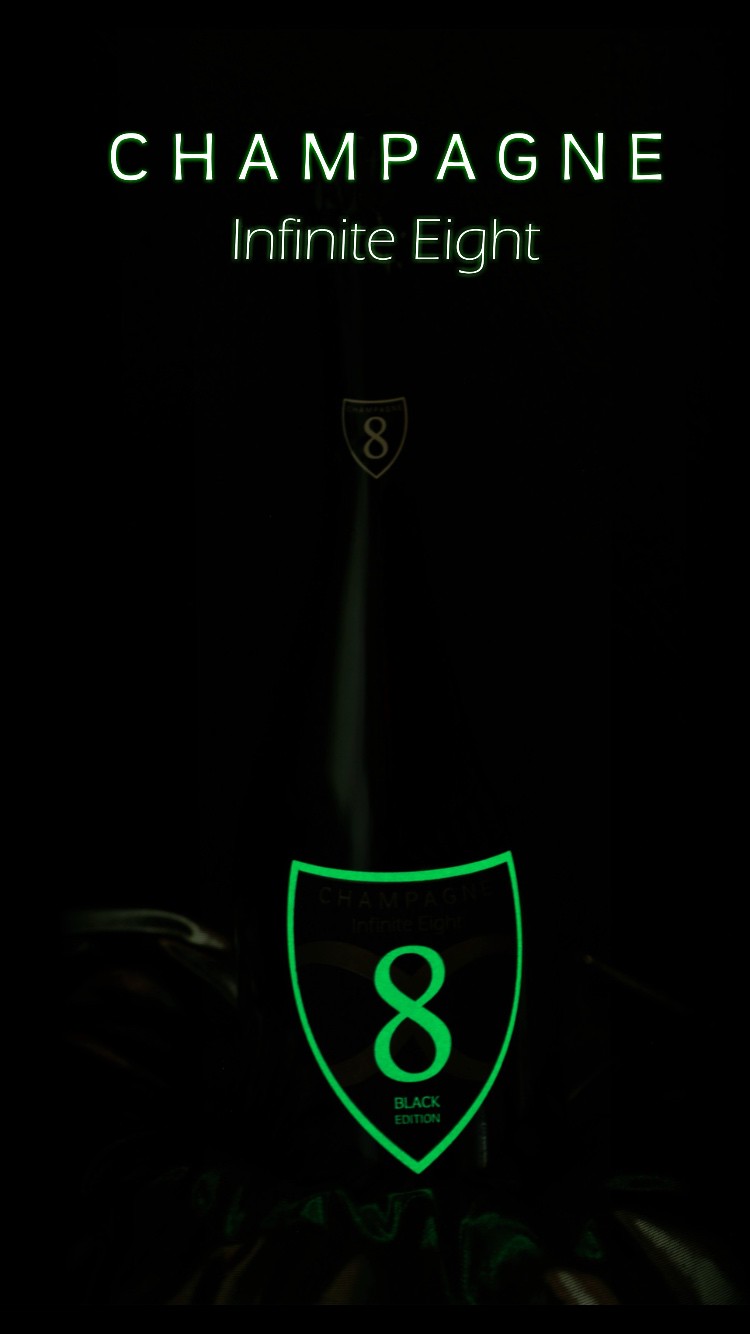This advertisement for a champagne brand features a predominantly black background, creating a sleek and mysterious aesthetic. At the top, the word "Champagne" is written in bold, white letters, followed by "Infinite 8" in a similar white text. Central to the ad is a black champagne bottle, highlighted by an eye-catching lime green shield design on its label. The shield's outline is vividly green, framing a black interior that bears the number "8" in the same bright green color. Below the shield, the label reads "Black Edition," though finer print beneath it is too small to discern clearly. The neck of the bottle features a smaller version of this shield, but with a copper or gold hue replacing the green. The bottle rests on a softly folded, reflective, black or grey satin material, adding to the luxurious feel of the presentation. Subtle, almost imperceptible green designs are scattered faintly at the bottom of the image, enhancing the overall aesthetic without detracting from the primary focus on the champagne bottle and its sophisticated branding.